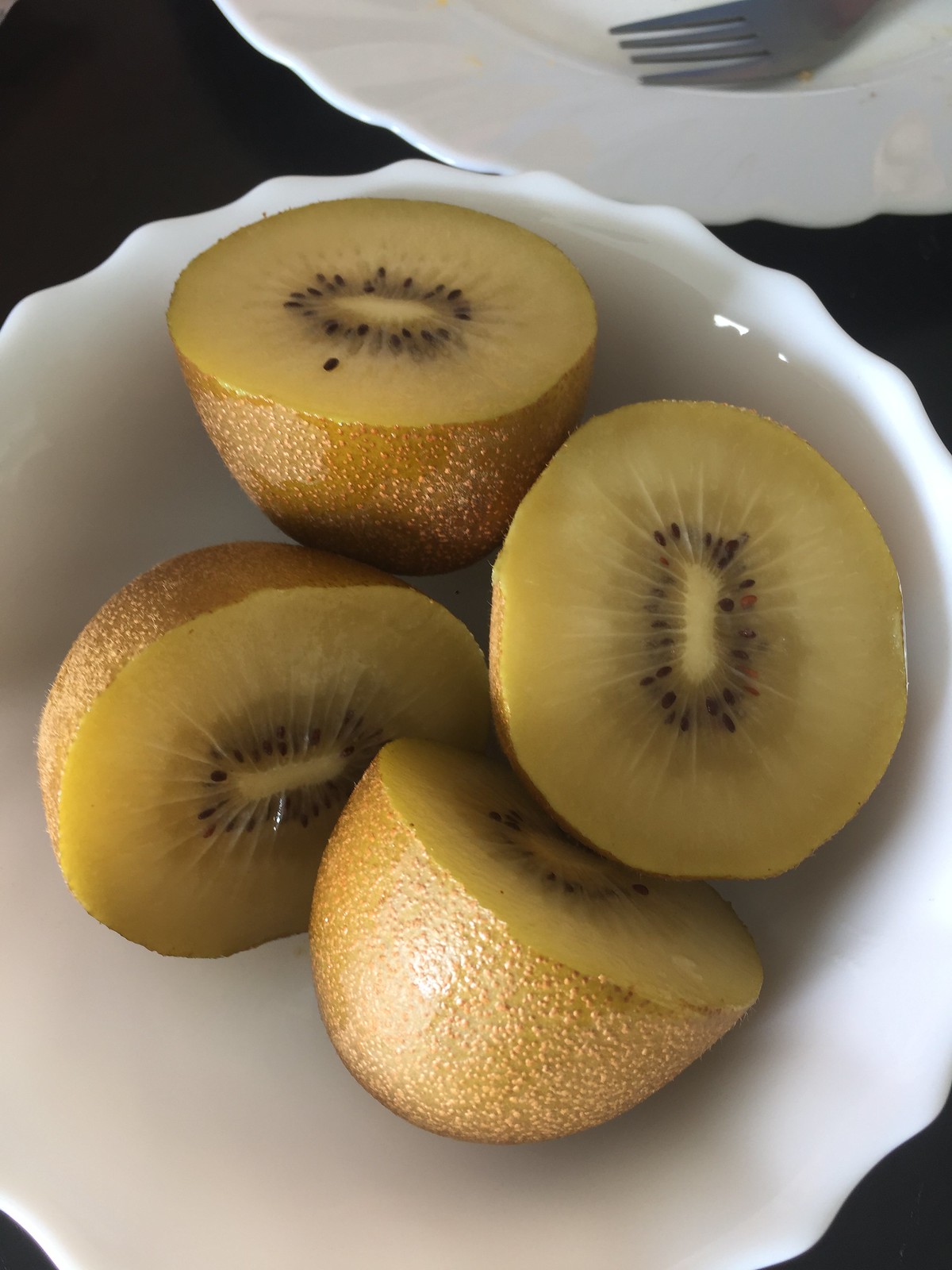A close-up image shows a white glass bowl with an irregularly shaped edge against a black background. Inside the bowl, four halves of kiwi fruit are arranged with their sliced sides facing the camera, revealing the dark olive green flesh. Each kiwi half features a thick white center surrounded by a radial pattern of small black seeds. The outer skin of the kiwis, visible on three halves, is brown with a tiny bumpy texture. Partially visible in the upper part of the photo is a white saucer with a four-pronged fork resting on it. The glossy surface of the bowl and the vibrant, freshly washed appearance of the kiwis make the colors and textures pop vividly against the dark background.